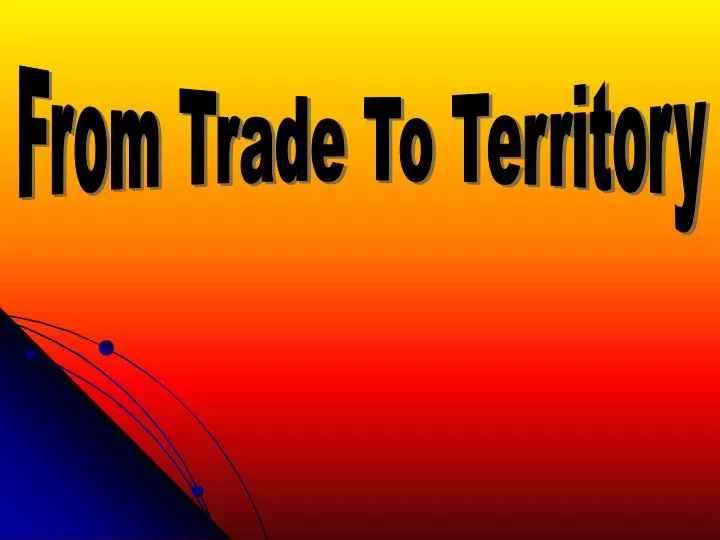The image depicts an early 2000s-style PowerPoint slide with a dated aesthetic. The background features a gradient transitioning from yellow at the top to dark red at the bottom, passing through shades of orange and bright red. Dominating the top of the slide is large, black text that reads "From Trade to Territory," with the lettering slightly wider at the edges and narrower in the center. In the bottom left corner, a dark blue triangle is positioned, showcasing its own gradient from a brighter to darker blue. Overlapping the triangle are several curvy lines, resembling orbits, each adorned with little blue dots, reminiscent of electrons circling an atom.